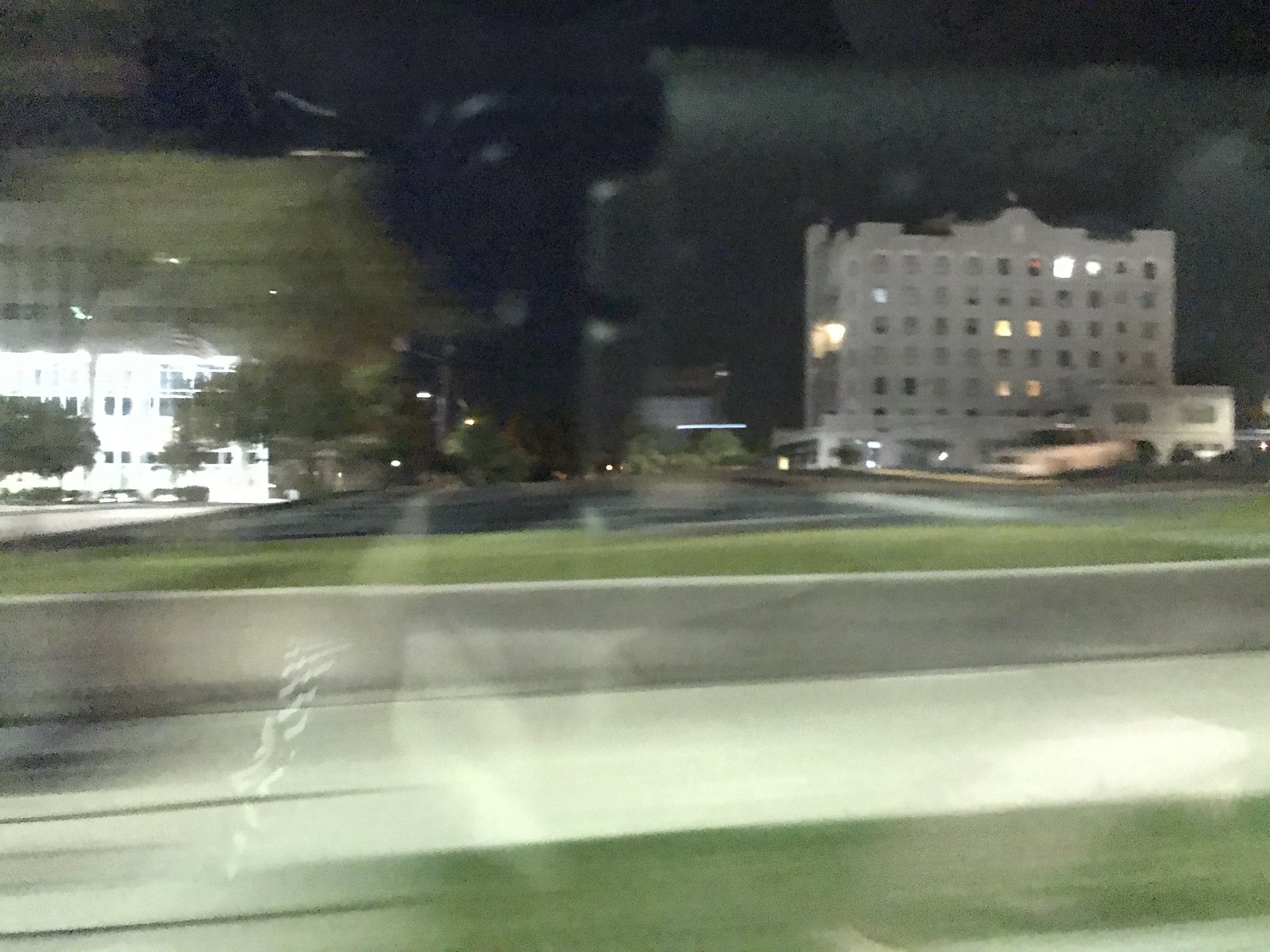This nighttime cityscape photograph, though slightly distorted and blurry, captures a lively urban setting with notable details. On the right side, a large, well-lit building with numerous windows dominates, fronted by a parking lot with a white taxi parked conspicuously. A road runs horizontally across the image, accompanied by a parallel sidewalk bordered by patches of grass. On the left, another white building stands out, illuminated brightly, suggesting artificial lighting that casts a fluorescent glow. Surrounding this building are several trees, adding a touch of greenery to the scene. The slight reflection present in the image hints that the photo might have been taken through a car window, contributing to its overall dreamy and surreal quality.